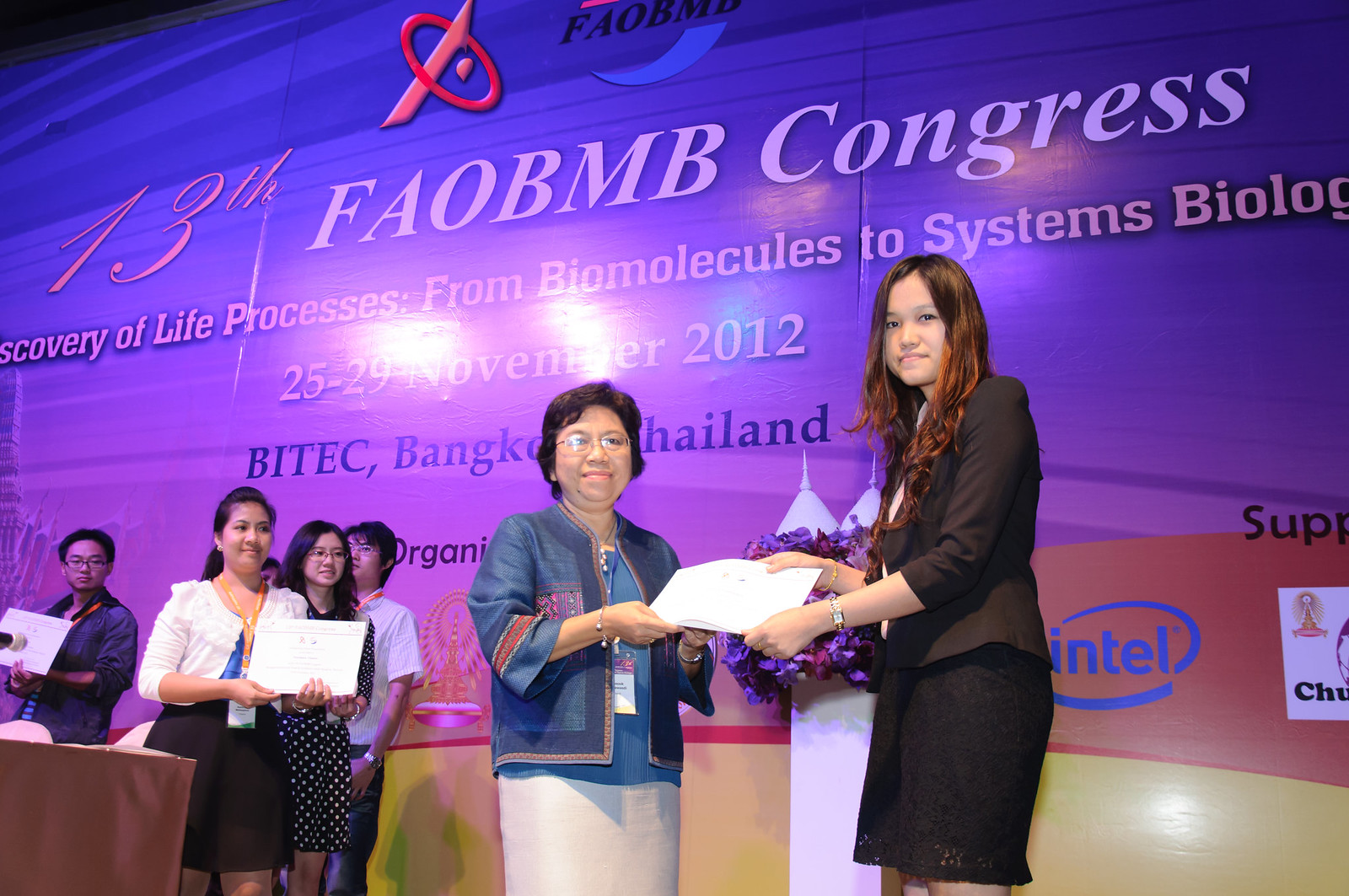The photograph captures an award ceremony at the 13th FAO BMB Congress, held from November 25-29, 2012, in Bangkok, Thailand. The focal point of the image is two women in the foreground, where an older woman with glasses and dark shoulder-length hair, dressed in a dark blue dress suit, is handing an award to a shorter woman wearing a blue dress shirt paired with a white long skirt. Behind them, four other young women are lined up, each holding plaques, indicative of their participation in the awards ceremony. The stage is set against a large blue banner with the inscription "13th FAO BMB Congress, Discovery of Life Processes from Biomolecules to Systems Biology." Logos, including those for Intel, are visible on the banner, reiterating the significance of the event.